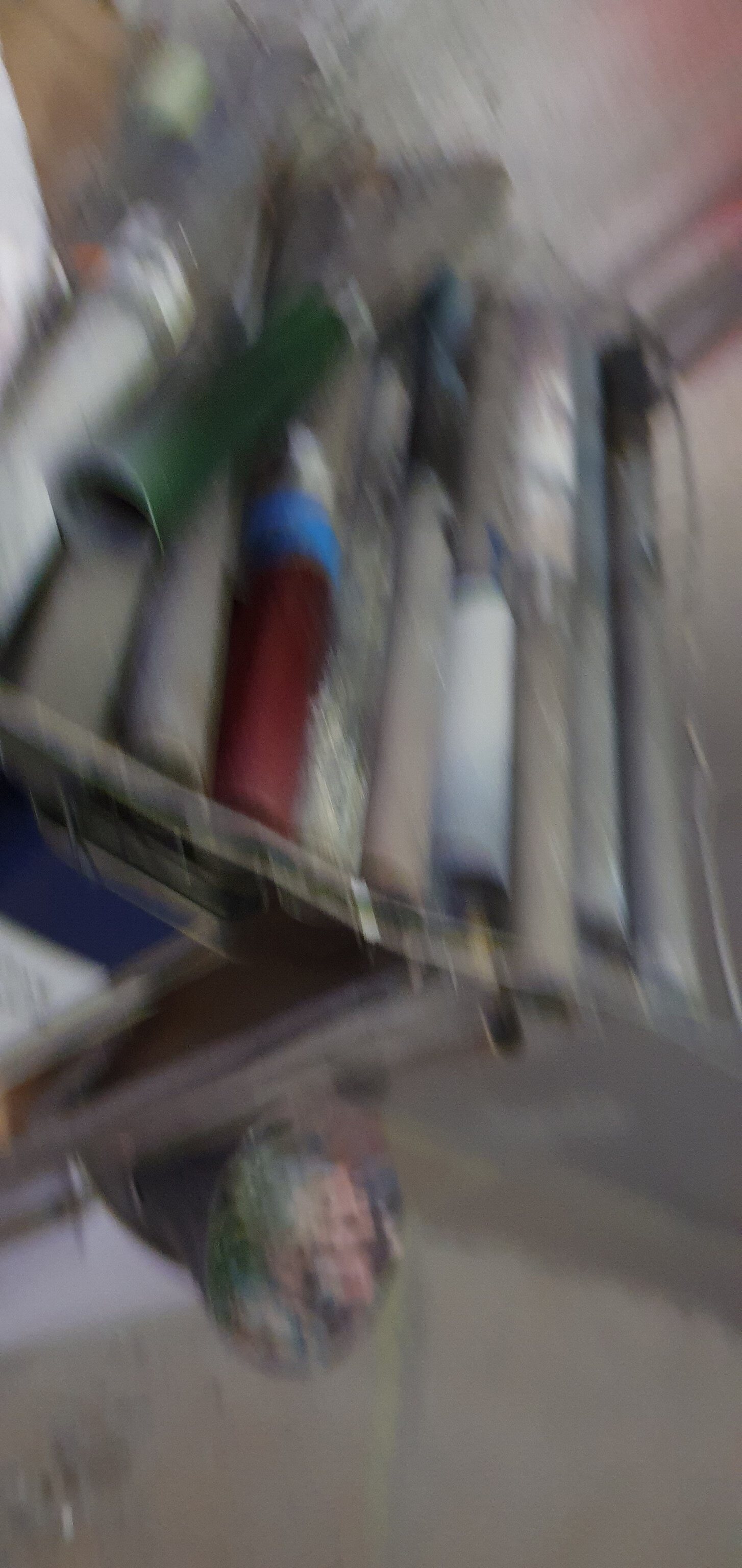The image is a blurry photograph focusing on a cluttered scene featuring a metal cart or table laden with various colorful tubes and handles. The handles, some appearing circular, are distinctly painted in green and red, with additional gray tubes flanking both sides. The items, possibly used for painting, are splattered with paint and add to the chaotic vibe of the scene. A notable blue stripe runs through the middle of these objects, though its purpose is unclear. The backdrop includes a white cement wall, and the gray-toned floor suggests a concrete or ceramic surface. Adjacent to the cart, there's what appears to be a wastebasket containing pink, light blue, and pale green items, possibly flowers.